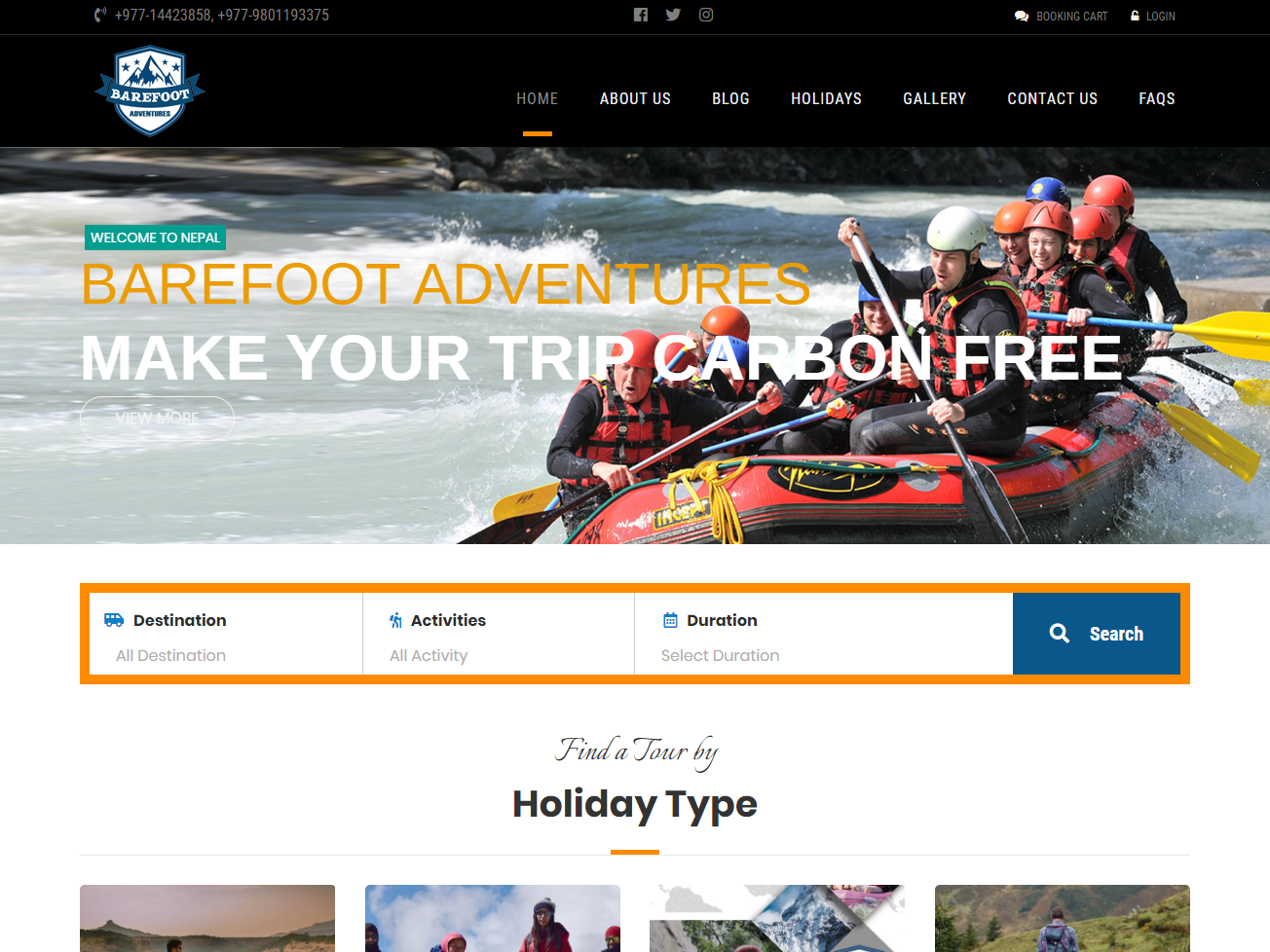The webpage showcases a striking layout with a black background at the top, featuring prominent social media icons for Facebook, Twitter, and Instagram. Positioned at the top right, the options for "Booking Cards" and "Login" are clearly visible. Below this, a series of navigation tabs are displayed: Home, About Us, Blog, Holidays, Gallery, Contact Us, and Fax, with "Home" highlighted and underscored by an orange line.

To the left, the site's logo, "Barefoot Adventures," is prominently positioned. The logo features blue hues, a mountain backdrop, and four blue stars. Centrally, the page welcomes visitors with "Welcome to Nepal, Barefoot Adventures" in prominent text. "Barefoot Adventures" is written in orange, while the tagline "Make Your Trip Carbon-Free" is in white, followed by a "View More" option. The background image shows people paddling a boat, donned in protective helmets—red, blue, and one white—and black protective swimwear along with yellow lifeguard vests. The boat itself is marked in yellow and black.

At the bottom, there's a section to set the destination, activities, and duration, alongside a blue search bar outlined in orange. This section is titled "Find a Tour by Holiday Type." Beneath this, various holiday pictures are displayed across the image. The background of the bottom part of the webpage is white, offering a clear and organized layout.